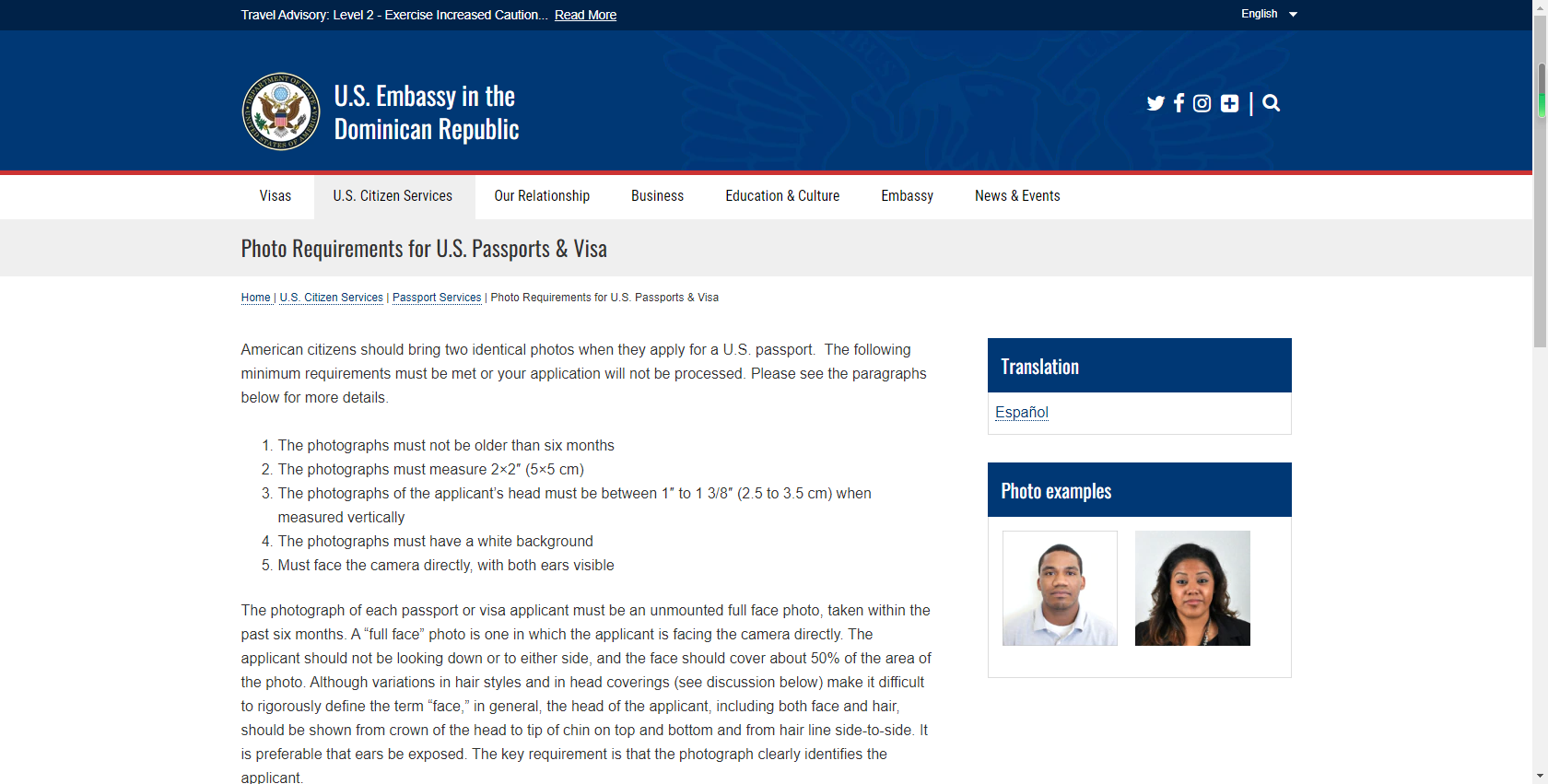This image is a detailed screenshot of the U.S. Embassy in the Dominican Republic's website, specifically the section outlining photo requirements for U.S. passports and visas.

At the top of the screenshot, there is a black bar highlighting a Travel Advisory Level 2, suggesting to "Exercise Increased Caution," followed by a "Read More" link. The interface also features a language selection drop-down menu set to English.

Centered on this bar is the emblem of the United States, featuring an eagle within a brown-and-white circle, and the text "United States Department of State" in black and white. To the right, "U.S. Embassy in the Dominican Republic" is displayed in white text against a blue background.

The upper right corner showcases icons for Twitter, Facebook, Instagram, Google+, a vertical line, and a magnifying glass search icon, all in white. Below this section is a bright red line, demarcating it from the rest of the content.

Immediately beneath, there is a navigation menu with headings including "Visas," "U.S. Citizen Services," "Our Relationship," "Business," "Education and Culture," "Embassy," and "News and Events." The current focus is on "Photo Requirements for U.S. Passports and Visas," nested under the "U.S. Citizen Services" tab.

The webpage details:

1. The photographs must be no older than six months.
2. Must measure 2x2 inches (5x5 cm).
3. The applicant's head must be between 1 inch and 1 3/8 inches (2.5 to 3.5 cm) measured vertically.
4. Photos must have a white background.
5. The applicant's face must directly face the camera, with both ears visible.

An additional paragraph elaborates on full-face photo requirements:
- Must show the applicant's head from the crown to the tip of the chin, and from hairline to hairline on the sides.
- The face should cover approximately 50% of the photo area.
- Eyes must be open and visible.
- Variations due to hairstyles or head coverings, which are elaborated on further in the document, should not obscure the face.

To the side of this text, there is a blue rectangle labeled "Translation" with a link to "Español." Below it, another blue rectangle reads "Photo Examples," showcasing compliant photos of a man and a woman with brown skin against white backgrounds.

This informative webpage from the U.S. Embassy provides clear and detailed guidelines for American citizens applying for passports and visas, ensuring their photos meet the necessary criteria.